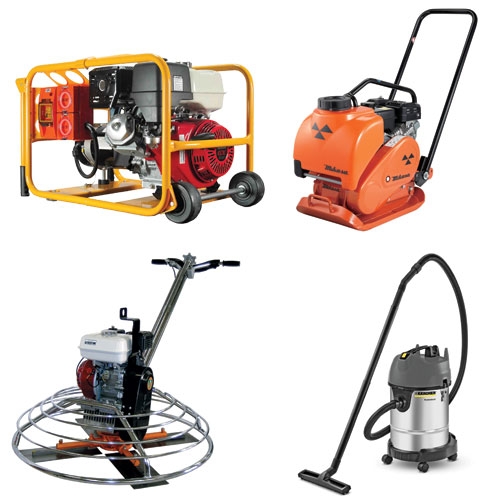The image displays four distinct outdoor power tools arranged in a 2x2 grid pattern against a bright and clear setting with excellent clarity. Each tool is presented in color, showcasing a palette that includes black, silver, red, yellow, and orange. 

In the top left corner, there is a red-and-yellow electric power generator equipped with a gray fuel tank and two wheels for portability. Adjacent to it, in the top right corner, is an orange soil compactor featuring three black triangular markings on its tank, a black fuel lid, and a sturdy black push bar. 

The bottom left corner houses an industrial floor sander or polisher, identified by its four rotating blades protected by a silver wire structure, a white plastic fuel tank, and a dual-handled black push bar. Lastly, the bottom right corner showcases a silver shop vacuum cleaner, complete with a black hose and a steel canister mounted on four wheels. The image employs a photo-realistic style, with backgrounds removed, allowing the tools to appear as if they are floating.